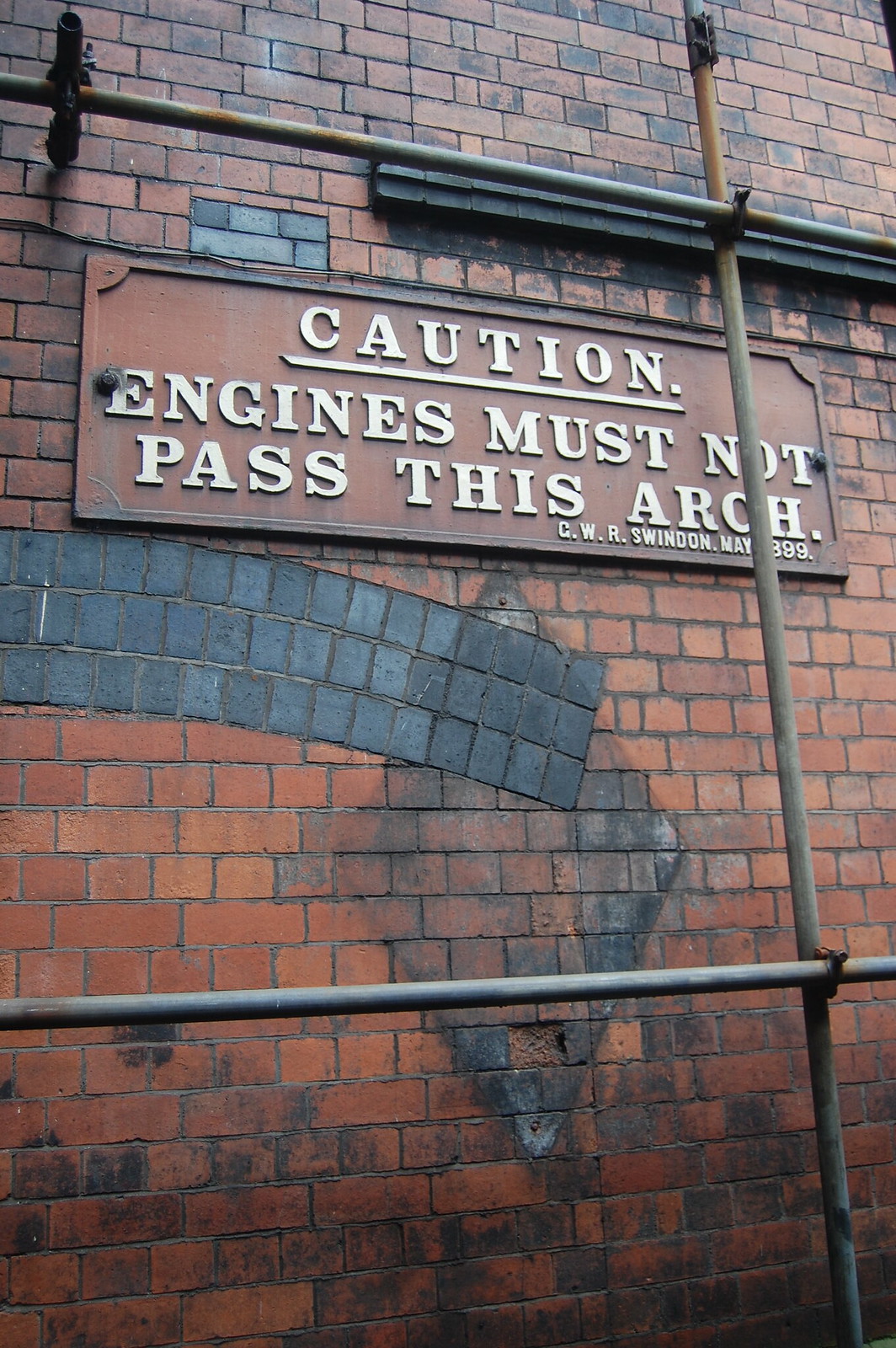The image shows the side of an old brick building with an affixed sign that reads, "CAUTION: Engines must not pass this arch." The sign appears to be made of reddish metal with white lettering and shows signs of wear. Above the sign, there's visible scaffolding suggesting ongoing construction or repairs. The brick wall itself has a mix of darker and lighter bricks arranged in an arc pattern, with some stains hinting at where an older sign might have been in a diagonal or diamond shape. White writing is also present, though largely overshadowed by the caution sign. Additionally, a few metal pipes traverse the image, zigzagging from the upper left to the bottom right, partially obscuring parts of the sign where a barely legible name, possibly "DWR Swenson," is written in small font. There are no figures, other colors, or additional signage in the picture, making the brick wall the central element.